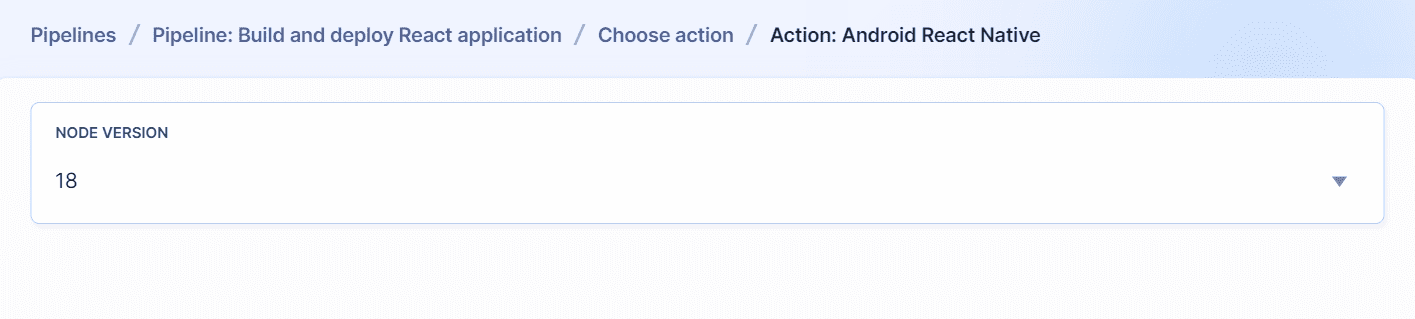The image in question is a wide rectangular format, approximately five to six times wider than it is tall. The top third of the image features a light blue background, while the bottom third has a white background. 

On the left side of the top section, there is black text that reads: "Pipelines / Pipeline: Build and Deploy React Application." All significant words have their first letter capitalized (Pipelines, Pipeline, Build, React).

Following this text, another forward slash leads to more instructions: "Choose Action / Action: Android React Native." Here, the words "Choose," "Action," "Android," "React," and "Native" also have their initial letters capitalized. This text spans about two-thirds of the top area.

Below this text, occupying the bottom two-thirds of the image, is a light blue-bordered rectangular box extending from left to right. Inside this box, the background is white. In the top-left corner of the box, "NODE VERSION" is written in all capital black letters. Toward the bottom left of this box, aligned to the left, the number "18" is displayed. In the lower right corner of the box, there is a black downward arrow, likely indicating an expandable menu for further options.